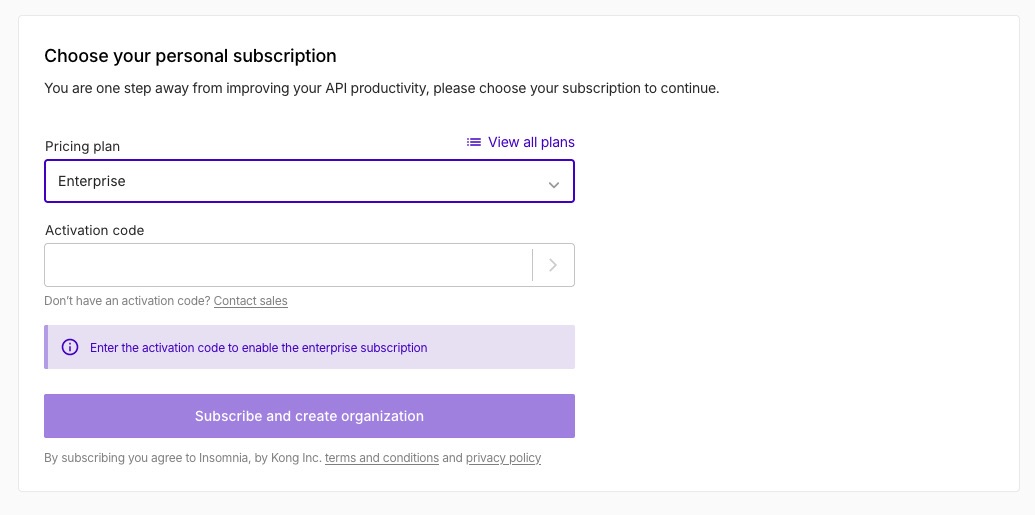This image is a cropped screenshot of a subscription sign-up page for an API service. Dominating the interface is a white box, bordered at the corners by a thin, grey outline. At the top of this box, in bold black font, the text reads "Choose Your Personal Subscription." Below this heading, there is a brief instruction: "You are one step away from improving your API productivity. Please choose your subscription to continue."

On the left side of the box, a label saying "Pricing Plan" is displayed, accompanied by a drop-down menu currently set to "Enterprise." On the right side, there is a hyperlink in purple labeled "View All Plans." Beneath this, in smaller black text, is the label "Activation Code," followed by a text box intended for users to input their code.

Just below the activation code text box, there is a prompt: "Don't have an activation code? Contact Sales," with "Contact Sales" being a clickable hyperlink.

At the bottom of the screenshot, a prominent purple banner instructs users to "Enter Activation Code to enable the Enterprise subscription." Below this banner is a large, darker purple button that reads "Subscribe and Create Organization." Finally, at the very bottom, a disclaimer states, "By subscribing you agree to Insomnia by Kong Inc. Terms and Conditions and Privacy Policy," with "Terms and Conditions" and "Privacy Policy" both serving as hyperlinks.